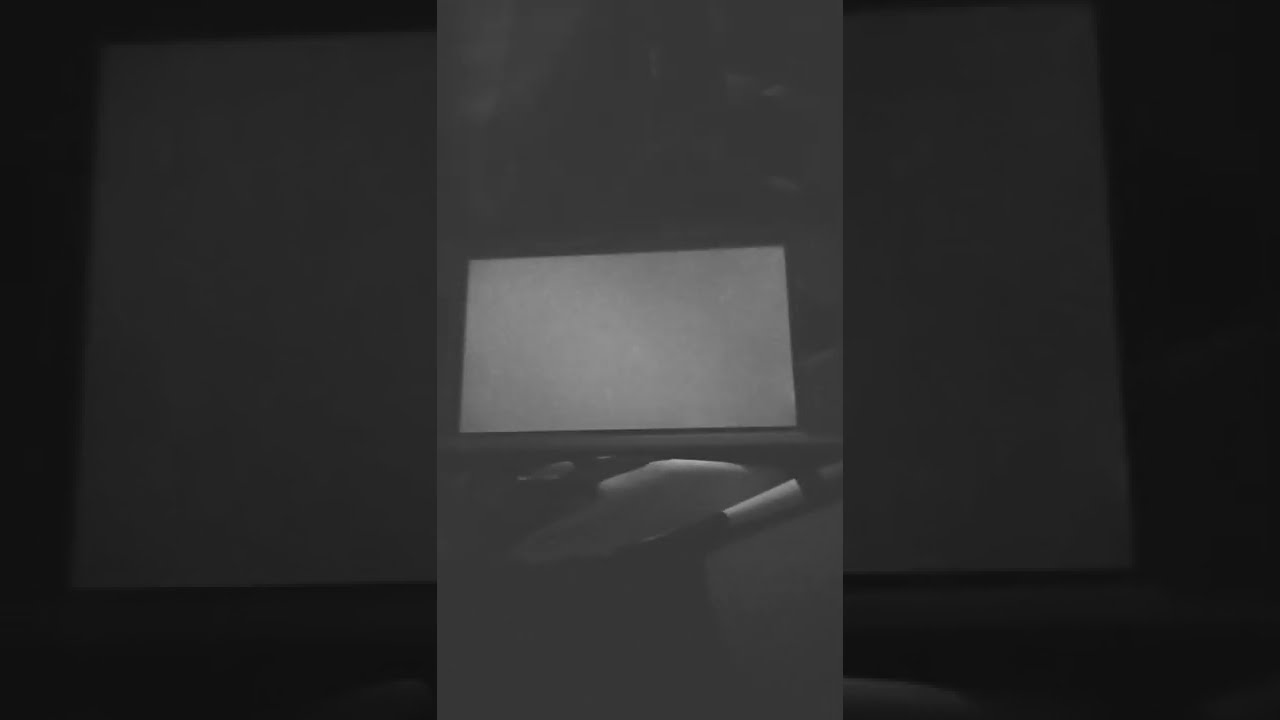This is a horizontally aligned black and white image with a centrally positioned white rectangular shape, which could potentially be a piece of paper, a folder, or an artist's white cardboard. The image features a dark background, primarily consisting of varying shades of gray and black. In the middle frame, there appears to be a silverish and black handle or possibly a paintbrush lying below the white rectangular shape, partially obscured by a nebulous dark object with a grayish surrounding. The image has a distinct division: the left section showcases a close-up view of the white board, and similarly, the right section offers a close-up of the right side of the board, both against a dark backdrop. The composition is somewhat abstract and out of context, making the precise identification of objects difficult, but the central white rectangle remains a clear focal point amid the predominantly grayed-out scene.